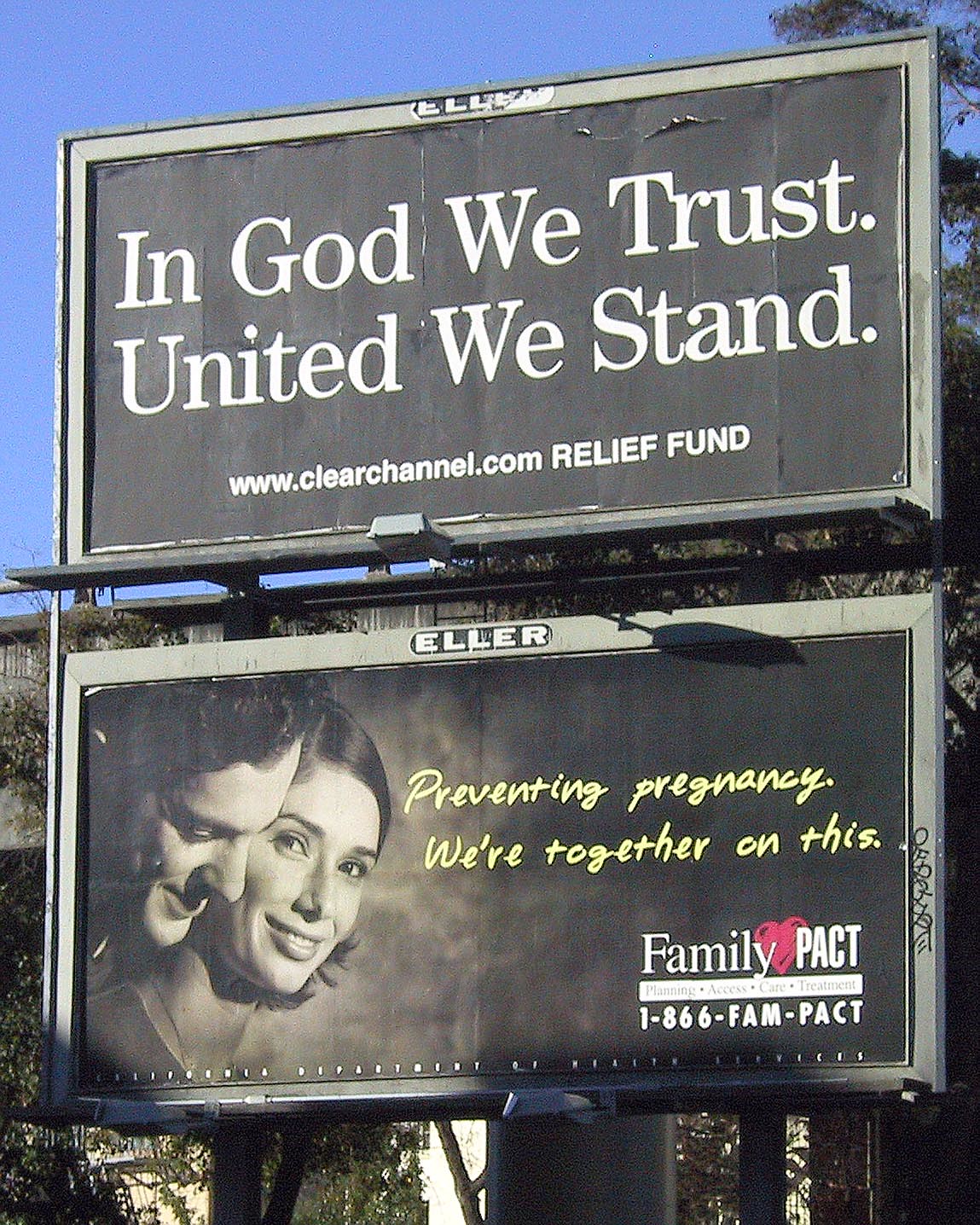This color photograph, taken outdoors, features two stacked billboards. The upper billboard has a black background with white text reading, "In God We Trust, United We Stand, www.clearchannel.com, Relief Fund." Below it, a second billboard starts with "Eller" in white lettering at the top. The main section of this lower billboard has a message in yellow text on a black background: "Preventing Pregnancy. We're Together On This." It also includes "Family PACT, 1-866-FAM-PACT, Planning Access Care and Treatment." The billboard displays a black-and-white image of a man looking over a woman's shoulder while she faces forward, staring ahead. The background at the top left of the image shows a clear blue sky, with trees and shrubs visible behind the billboards.